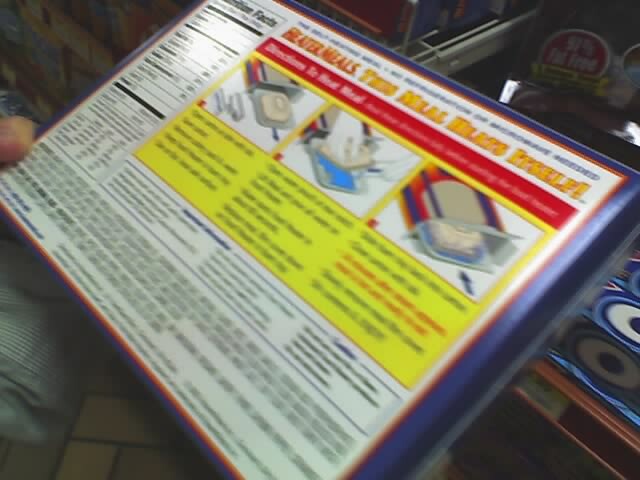The image depicts the back of a product label, partially obscured and slightly blurred. The label appears to provide step-by-step instructions for preparing a meal, divided into three distinct sections. In the first section, an illustration shows the box being opened. The second section depicts an item being taken out of the box and something being placed on it, likely indicating an additional ingredient or a preparation step. The final section shows the item being returned to the box, possibly for heating or final preparation.

To the left of the instructions, there seems to be a nutritional facts panel, although the specifics are unreadable due to the blur. This panel extends vertically and includes detailed information that occupies the entire length of the label. At the bottom of the label, additional textual information is visible but similarly indistinct. Someone is holding the box, which partially obstructs the view, but the overall setup suggests it is designed to guide the user through the meal preparation process.